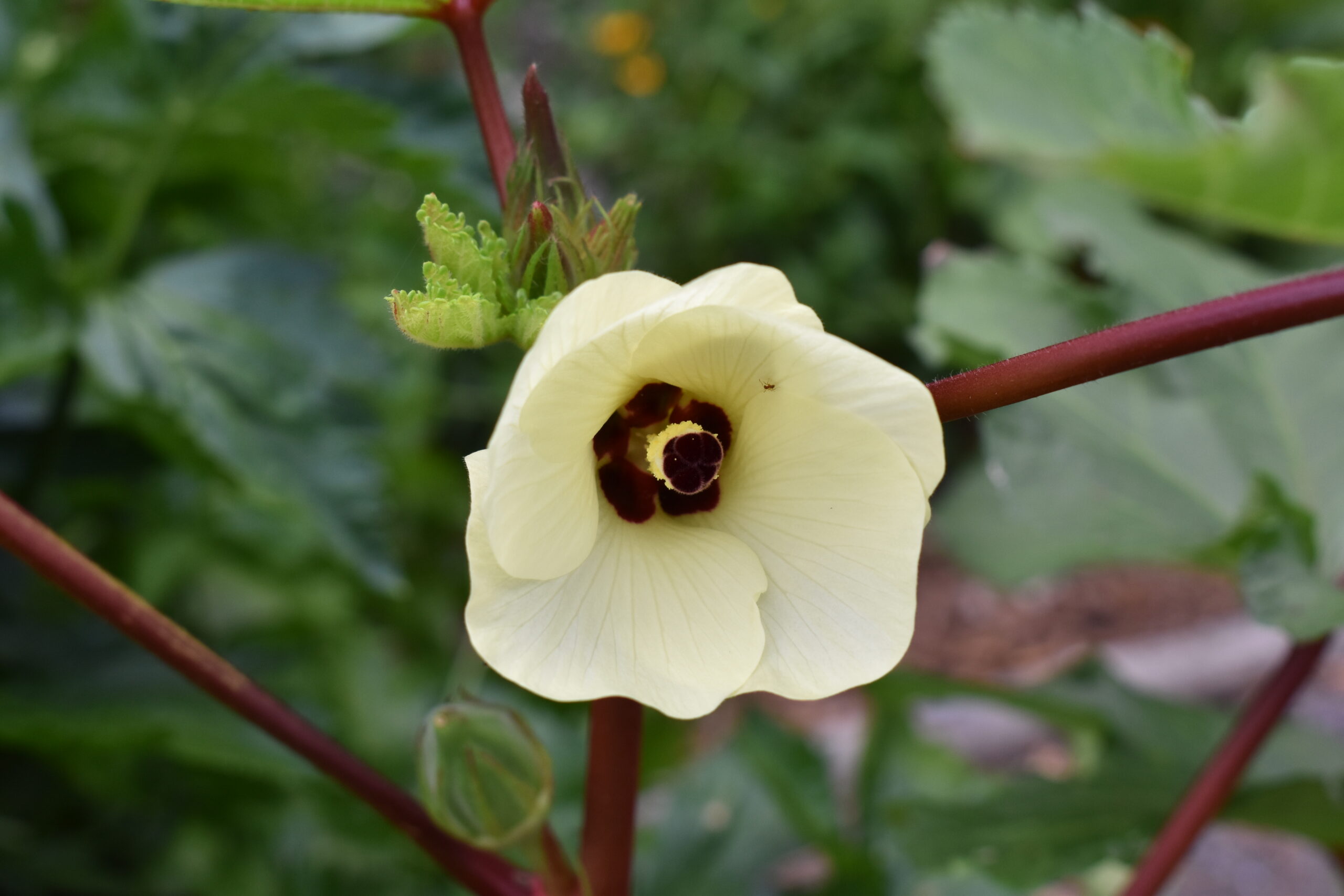The image is a close-up shot of a white flower displaying a rich blend of yellow and brown in its center, with distinctive black stamens and black pollinators nestled inside. The scene is set against a backdrop of blurred, lush green leaves, with an apparent bokeh effect that softens the details in the background. The stem or branches supporting the flower are reddish-brown, adorned with additional green buds and leaves. The petals of the flower feature subtle grayish lines, and there's a small bug visible crawling inside the flower. Bright sunlight casts shadows and highlights on the flower, suggesting it was taken on a sunny day. The overall composition emphasizes the vibrant contrasts and intricate details of the flower while maintaining a soft, unfocused green background.